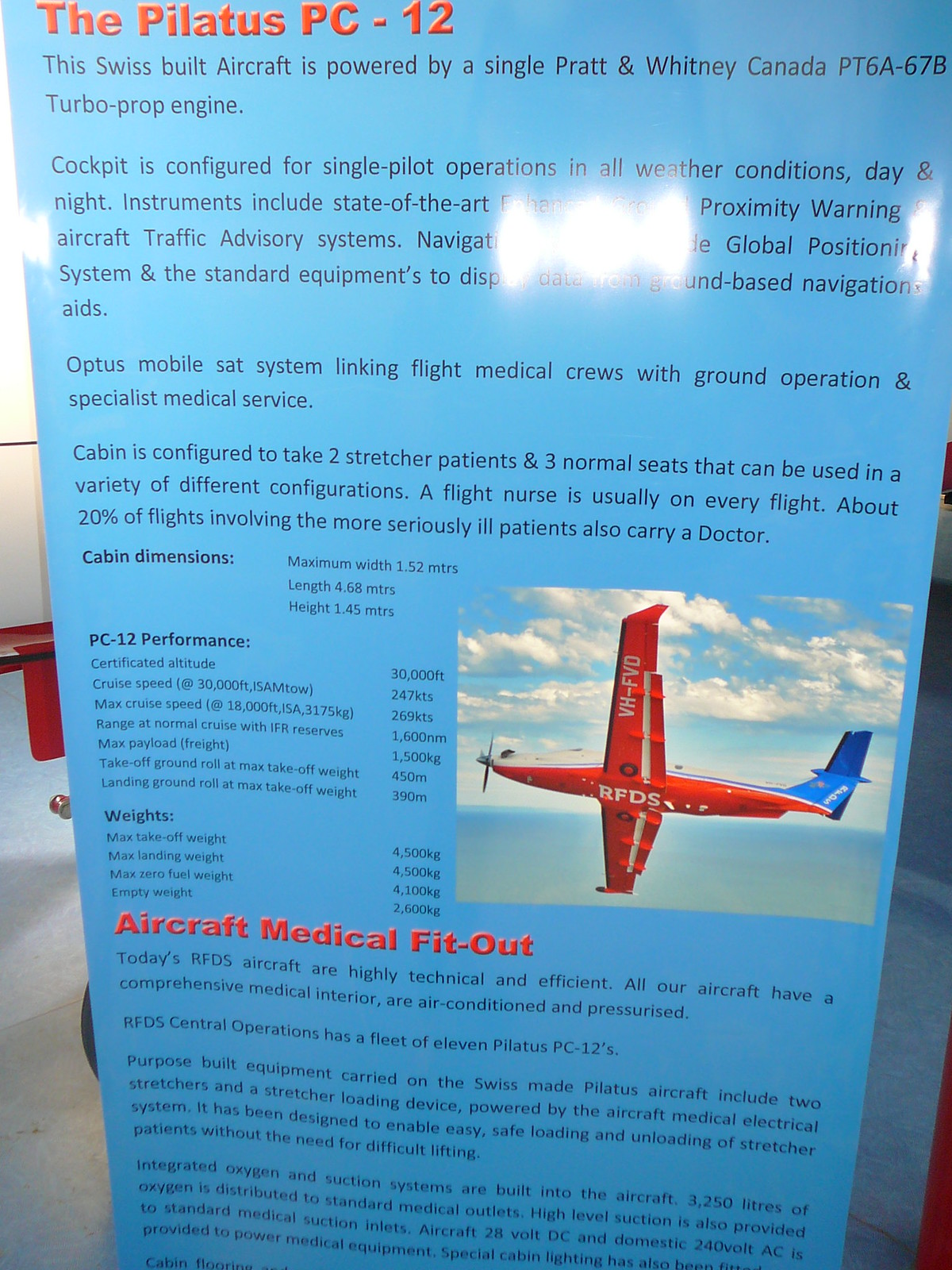The image features an educational poster detailing the Pilatus PC-12, a Swiss-built medical aircraft prominently highlighted in the center. The poster showcases the airplane depicted in red with a white stripe and a blue tail, prominently situated in the lower right half of the image, with markings "RDS" on the body and "WH FBD" on the wing. The aircraft is powered by a single Pratt & Whitney Canada PT6A-67B turboprop engine and is designed for single-pilot operations in all weather conditions, day and night. The cockpit is equipped with advanced proximity warning systems, aircraft traffic advisory systems, a sophisticated navigation global positioning system, and standard instruments for ground-based navigation. The medical configuration of the cabin allows for two stretcher patients and three regular seats, accommodating various medical and operational needs. Additionally, around 20% of flights with seriously ill patients also include a doctor. Detailed performance statistics including maximum altitude, weight, and cabin dimensions are provided. This descriptive poster uses a palette of gray, black, white, red, light blue, and dark red, and emphasizes the medical capabilities of the aircraft, reinforcing its purpose with specific details about its configuration and equipment.